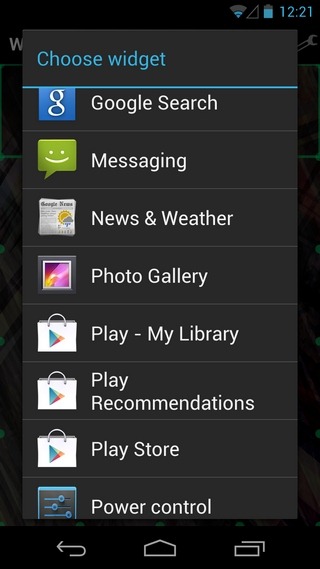This is a screenshot of a widget selection menu on a mobile device. The interface features a dark gray background, with a light blue header displaying the text "Choose Widget." A blue dividing line separates this header from the main content below. The menu showcases several widgets, each accompanied by an icon on the left and descriptive text on the right. The widget options include Google Search, Messaging, News and Weather, Photo Gallery, Play My Library, Play Recommendations, Play Store, and Power Control, all separated by thin light gray lines. This widget selection screen occupies most of the phone display. The bottom of the screen shows the phone's navigation buttons: Back, Home, and Menu. At the top of the screen, the phone's status bar is visible, indicating the signal strength, Wi-Fi connection, battery life, and the current time, which is 12:21.